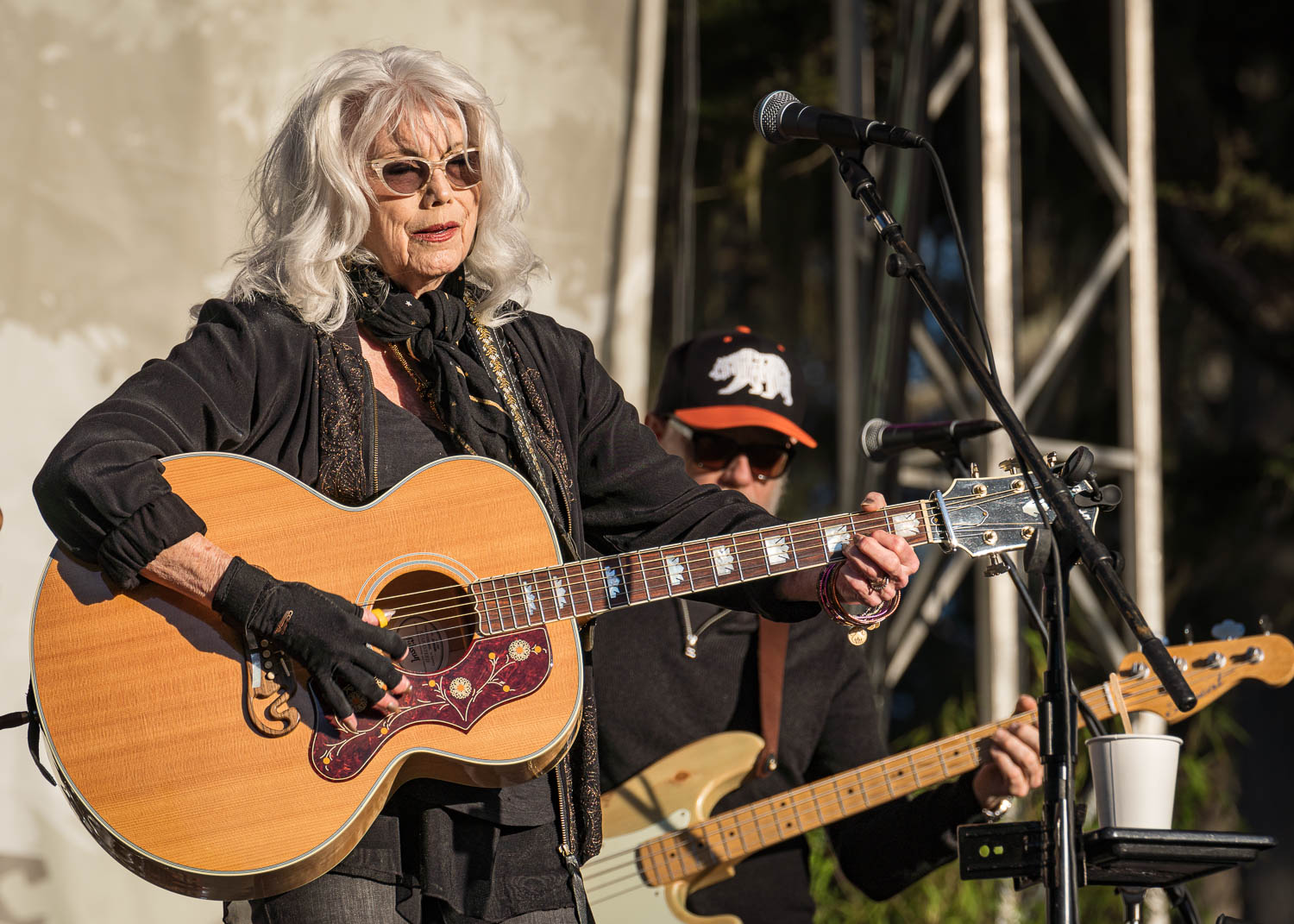In this detailed image, we see Emmylou Harris passionately performing on stage at a concert or music festival. She is dressed entirely in black, wearing a black jacket with a bit of glitter at the center, a black shirt, black pants, and a black scarf around her neck. Her shoulder-length white hair contrasts with her peach or pink-rimmed sunglasses, which are tinted but not overly dark, allowing a glimpse of her eyes. She has dark red lipstick on, adding a vibrant touch to her appearance. 

Emmylou is playing an acoustic guitar adorned with floral designs around the strings area. Her right hand, which is strumming the guitar, is gloved in a black fingerless glove, while her left hand, which holds the neck of the guitar, is decorated with multiple bracelets and possibly brownish fake nails. In front of her is a microphone into which she is singing. 

Behind her to the right stands a man playing an electric guitar. He is dressed in a black long-sleeve shirt and a hat featuring a polar bear design, reminiscent of the California state flag, with the tip of the hat colored in an orangey-red hue. He also wears sunglasses and a necklace over his shirt. There is another microphone set up for him. The setting gives off a warm, engaging atmosphere, capturing a beautiful moment of live music performance.